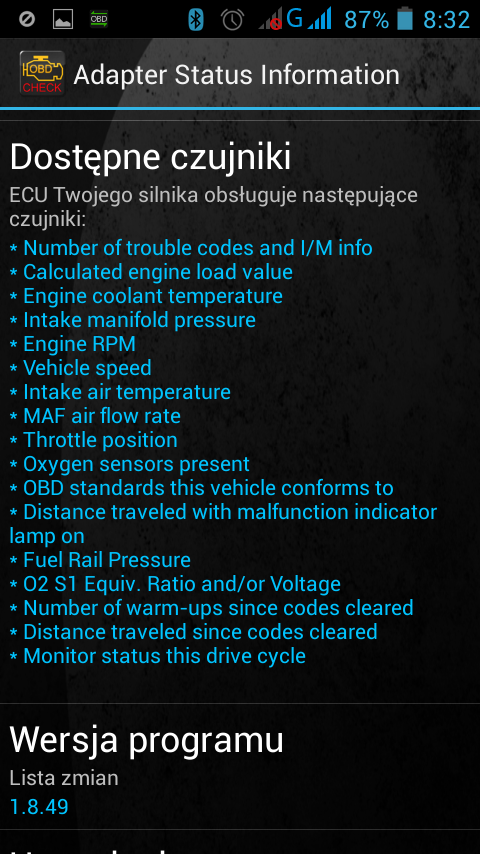The image is a detailed screenshot taken from an Android mobile device, showing an app interface. The app is likely related to vehicle diagnostics, as indicated by the content and terminology used throughout the screenshot. The top part of the display includes standard mobile status icons such as cell phone bars, battery percentage at 87%, and the time indicated as 8:32.

Below these icons, the app interface starts with the title "Adapter Status Information" in white text. The section underneath is filled with detailed diagnostic information presented in light blue text against a black background. The entries are organized in a bulleted list format, though instead of traditional bullet points, small stars are used. The listed items include metrics such as "Number of Trouble Codes and IM Info," "Calculated Engine Load Value," "Engine Coolant Temperature," "Intake Manifold Pressure," "Engine RPM," "Vehicle Speed," "Intake Air Temperature," "MAF Air Flow Rate," "Throttle Position," "Oxygen Sensors Present," "OBD Standards This Vehicle Conforms To," "Distance Traveled with Malfunction Indicator Lamp On," "Fuel Rail Pressure," "Zero to S1 EQIV Ratio and/or Voltage," "Number of Warmups Since Codes Cleared," "Distance Traveled Since Codes Cleared," and "Monitored Status This Drive Cycle."

Toward the bottom of the screenshot, there are two lines of text in a foreign language, possibly Central European, characterized by words such as "WERSJA PROGRAMU" and "Lista Zmijan." The numbers "1.8.49" are also visible. The overall color scheme of the screenshot includes black, white, gray, light blue, green, yellow, and red.